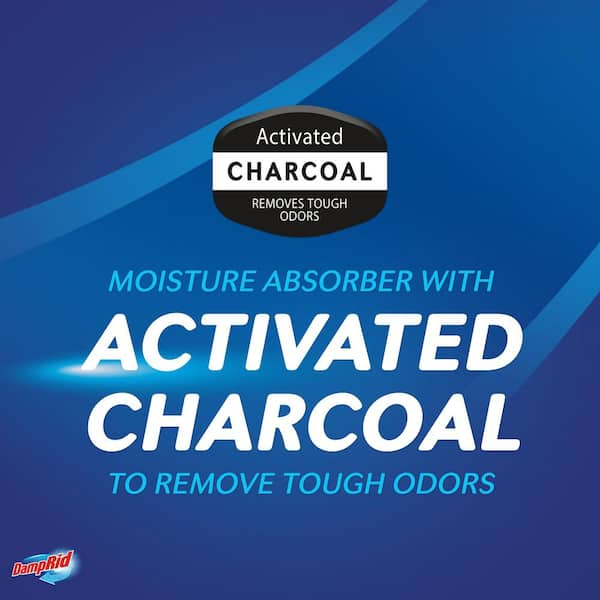This advertisement for DampRid prominently features a detailed design emphasizing its moisture-absorbing and odor-removing capabilities. At the top center, an oblong shape contains the phrase "activated charcoal removes tough odors," with the text in alternating black and white to match its background. Beneath this, in large white lettering, "activated charcoal" is displayed boldly, highlighting the key ingredient. Below it, in light blue letters, the text reads, "to remove tough odors," reinforcing the product's function. The main background has a blue square with light blue curved stripes flowing from right to left. Situated at the bottom left corner is the DampRid logo, marked by red letters with a curved blue arrow pointing left. Overall, this advertisement underscores the combination of a moisture absorber with activated charcoal to effectively combat persistent odors, making it ideal for use in areas like garages and basements.